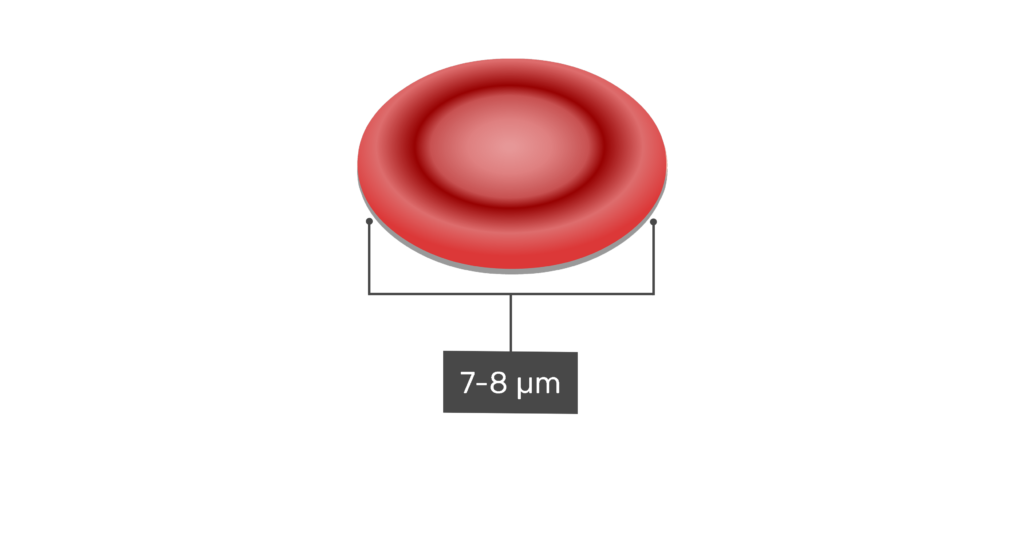The image displays a drawing of a rosy-colored, circular object resembling a blood platelet or a rubber seal, characterized by a distinct dark maroon ring around its perimeter. The circle has a central lighter area fading to almost white. This object could be perceived as a machinery part, potentially a rubber seal, with a donut-like shape and a flat center that raises around the edges, giving each edge a height of approximately half an inch. The background is plain white with no visible borders. Below the object are measurement lines indicating its dimensions. These lines converge into a single vertical line connected to a dark gray rectangle at the bottom, displaying the measurement "7-8 UM" in white print with the 'U' symbol resembling a 'P' without its upper part.